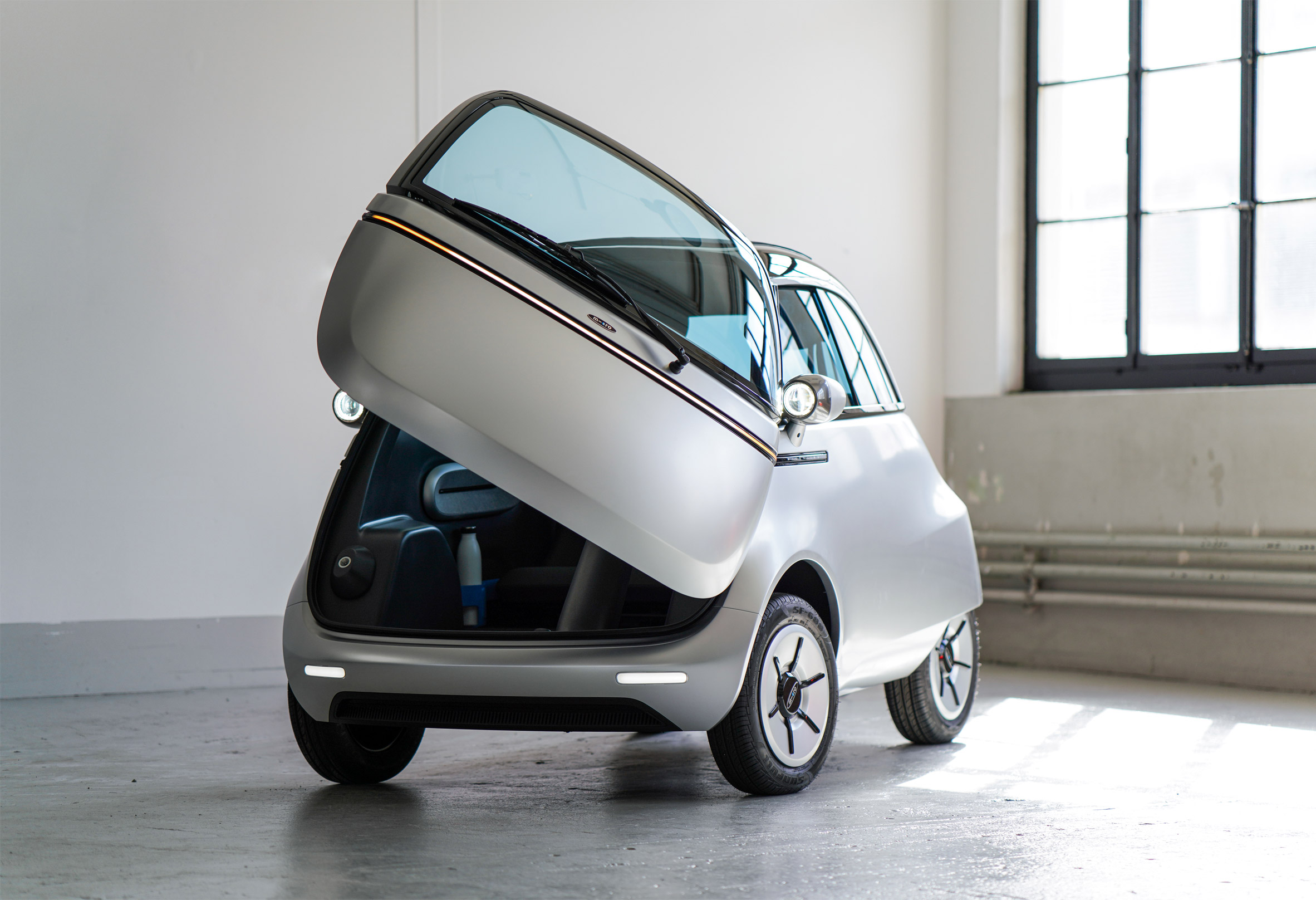In the image, a tiny, ultra-modern silver car is the centerpiece, situated in a spacious garage. The car resembles a smart car or a very compact, rounded vehicle without sharp angles, reminiscent of a VW Beetle but even smaller. Its strikingly futuristic design is accentuated by the unconventional way its front hood—or what might be the trunk—opens upward and towards the side, revealing some storage space behind it. The lack of visible writing or text on the vehicle adds to its sleek, minimalist appearance. The garage itself has white concrete walls and a medium-gray painted floor, with a large black-framed window on the right side that floods the room with natural light. This open window, along with the overall modern aesthetic of the car and interior, contributes to a bright, high-tech atmosphere.